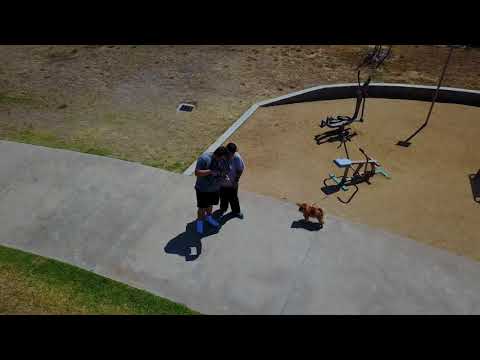In this top-down, somewhat blurry photograph taken from a high perspective, possibly by a security camera, two men stand closely together on a wide, grey paved walkway in a dry, park-like setting. The men are looking downward, seemingly focused on something one of them is holding, likely a cell phone. Nearby, a small brown dog stands at their side. The image features a mix of environments: a sandy area with playground-like equipment bordered by concrete to the upper right, patches of lush green grass, and expanses of dry, dying grass indicative of late summer circumstances. A drainage gate is also visible behind the men, adding to the sense of a public park or pathway.